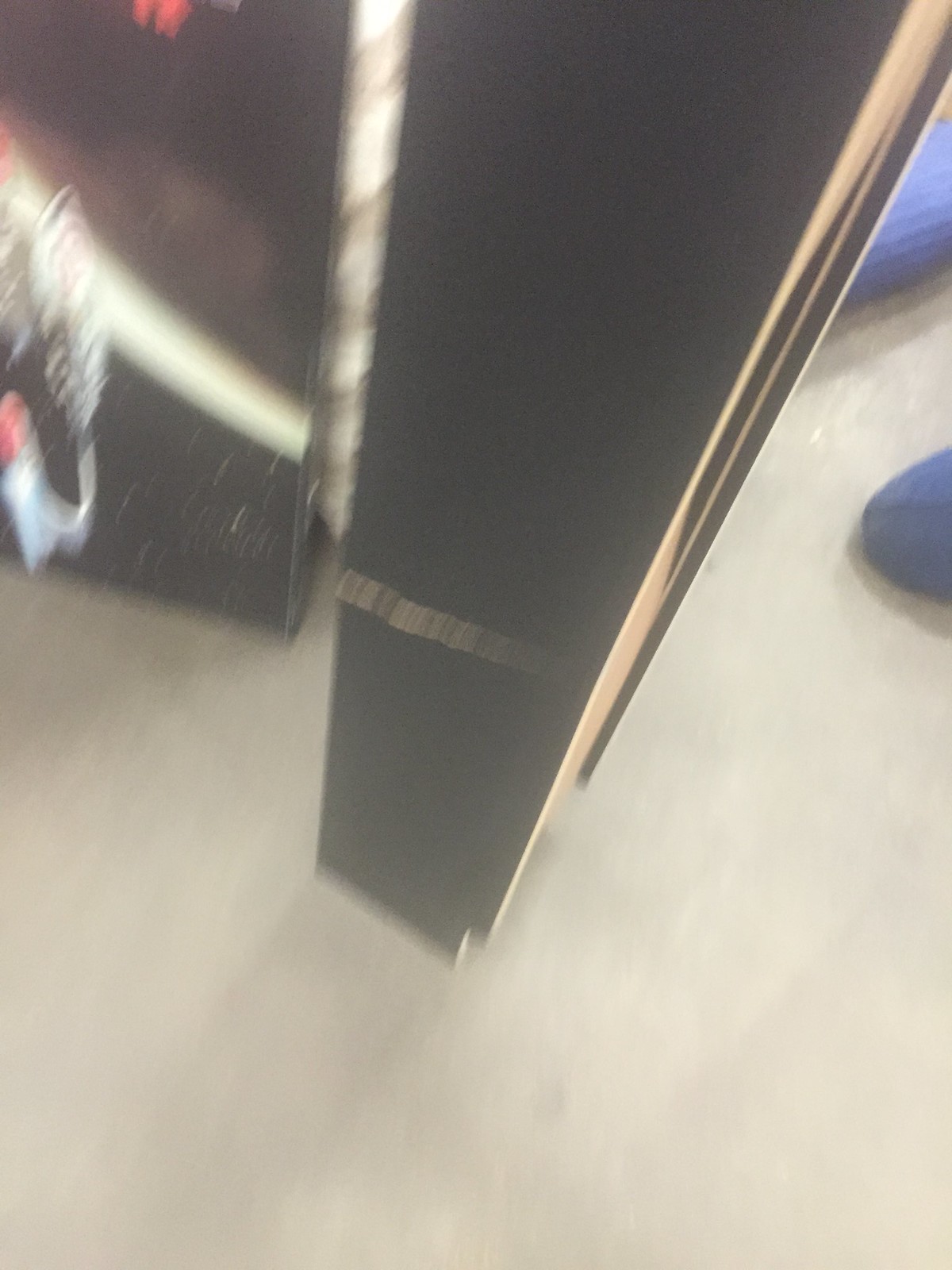The image captures a slightly blurry photograph, suggesting movement from the person who took it. The scene appears to be inside a store or shopping department, though context clues are minimal. At the center of the image stands a black pole, set in the middle of a walking area. To the left of the pole, there's a large painting resting on what seem to be containers. The painting has a dark, black background with a white strip running through its center, resembling a depiction of the galaxy with scattered stars. The overall image quality is not high definition, contributing to a sense of motion in the photo.